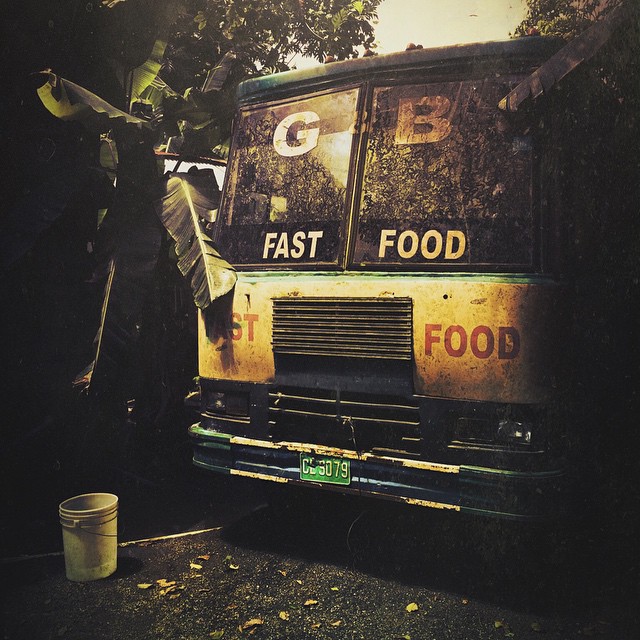The photograph depicts the front of a large, old vehicle, possibly a bus or van, parked outdoors in a dimly lit area. The vehicle, which appears dirty and neglected with debris on the ground and foliage hanging over it, highlights a sense of abandonment. On the windshield, the letters "G" and "B" stand out on either side, accompanied by the words "fast food" prominently displayed. Below the windshield, on either side of the front grille, the phrase "fast food" appears again in bold, red letters. The vehicle's green license plate, marked "CL-9079," is positioned beneath the front bumper, alongside visible headlights. A noticeable white bucket lies on the ground to the left of the vehicle, adding to the cluttered and overgrown scene that suggests the vehicle has been stationary for some time. The image, characterized by its graininess and dim lighting, perhaps due to editing or natural conditions, gives off a vintage or sepia-toned effect, enhancing the sense of timeworn abandonment.